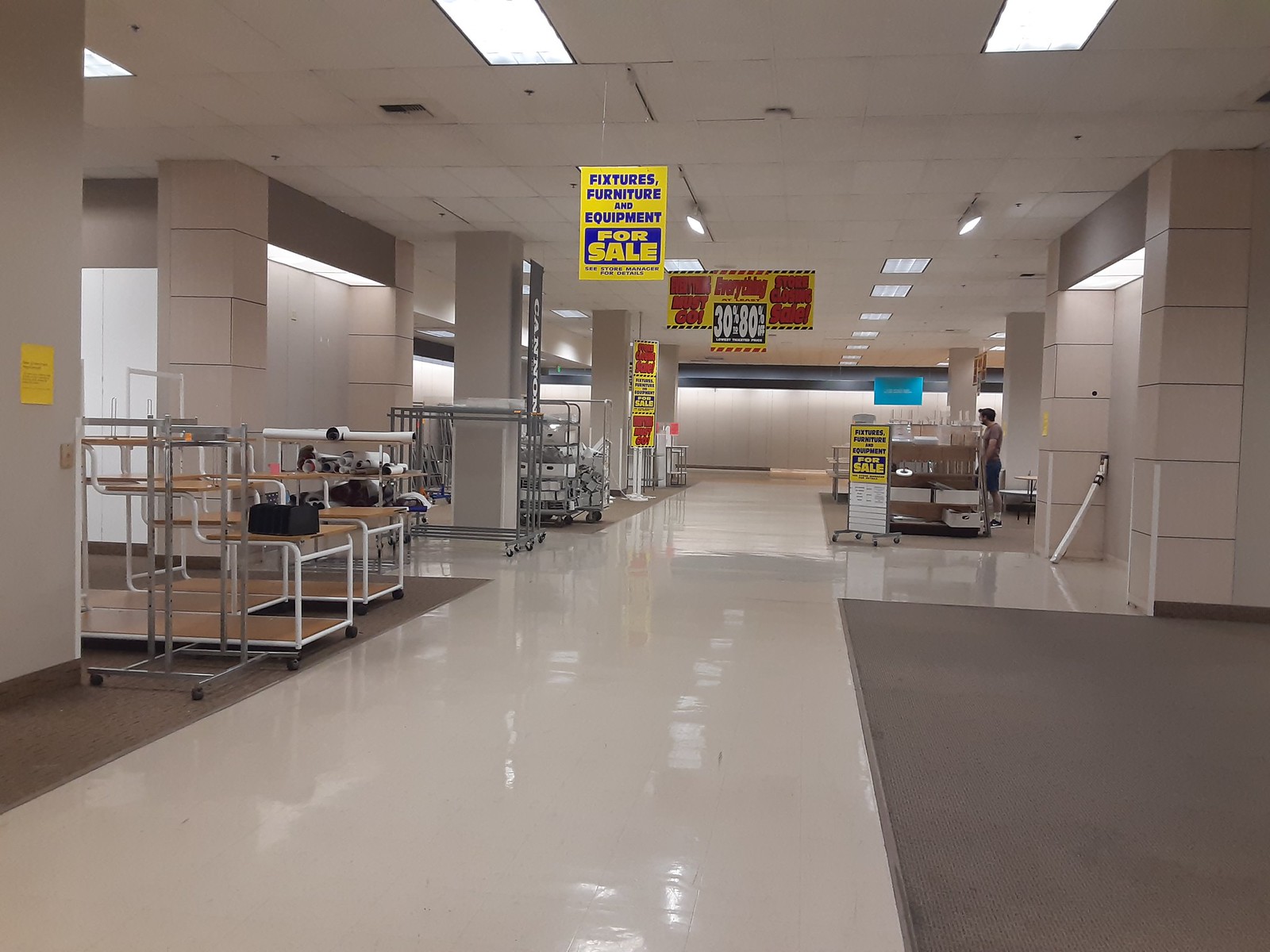In this image, we see a large store aisle characterized by its white walls, floors, and ceilings, all brightly illuminated by numerous ceiling lights. The aisle has gray carpeting along either side, providing a subtle contrast to the overall whiteness. Several rolling shelves are scattered throughout the aisle, sparsely occupied by remaining merchandise. Prominent, colorful signs draw attention: large yellow signs with blue letters advertise "Fixtures, Furniture, and Equipment for Sale," and bold red print on other yellow signs announce discounts ranging from 30% to 80% off. In the background, a blue sign adds to the visual noise. The sparsely filled shelves and the abundance of discount signs convey a sense of emptiness and impending closure, giving the store a rather melancholic ambiance.